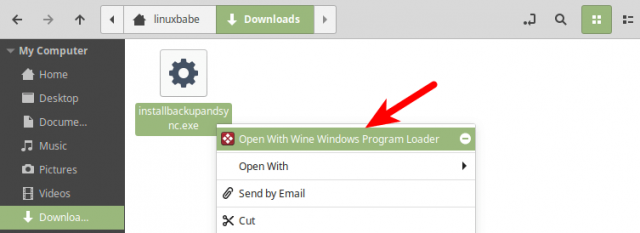The screenshot depicts a computer program interface with a medium gray header at the top. The header features a series of boxed arrows and options, most of them in gray boxes. Starting from the left, the first box contains a left-pointing arrow. To its right is a wider box with a gray house logo labeled "Linux Babe." Following this, there is a box in sand green displaying white text that says "Downloads" accompanied by a white, downward-pointing arrow. Next in line is another box that contains a right-pointing arrow.

Beneath the header, on the left side, there is a gray sidebar. At the top of the sidebar, "My Computer" is written in white text. Below this, there are several sections, each with a white icon and label: a house icon labeled "Home," a box labeled "Desktop," a paper icon labeled "Documents," an eighth note labeled "Music," a camera labeled "Pictures," a filmstrip labeled "Videos," and an arrow pointing down labeled "Downloads."

The main section of the screenshot, taking up the bulk of the page, has a white background. In the top left of this area, there is a file icon. The icon is a light gray box with a thin medium gray outline, rounded corners, and a dark gray cog symbol in the middle. Below the icon, highlighted in sand green with white text, is the filename "install_backup_and_sync.exe." A right-click context menu is open, with the top option labeled "Open with Wine Windows Program Launcher."